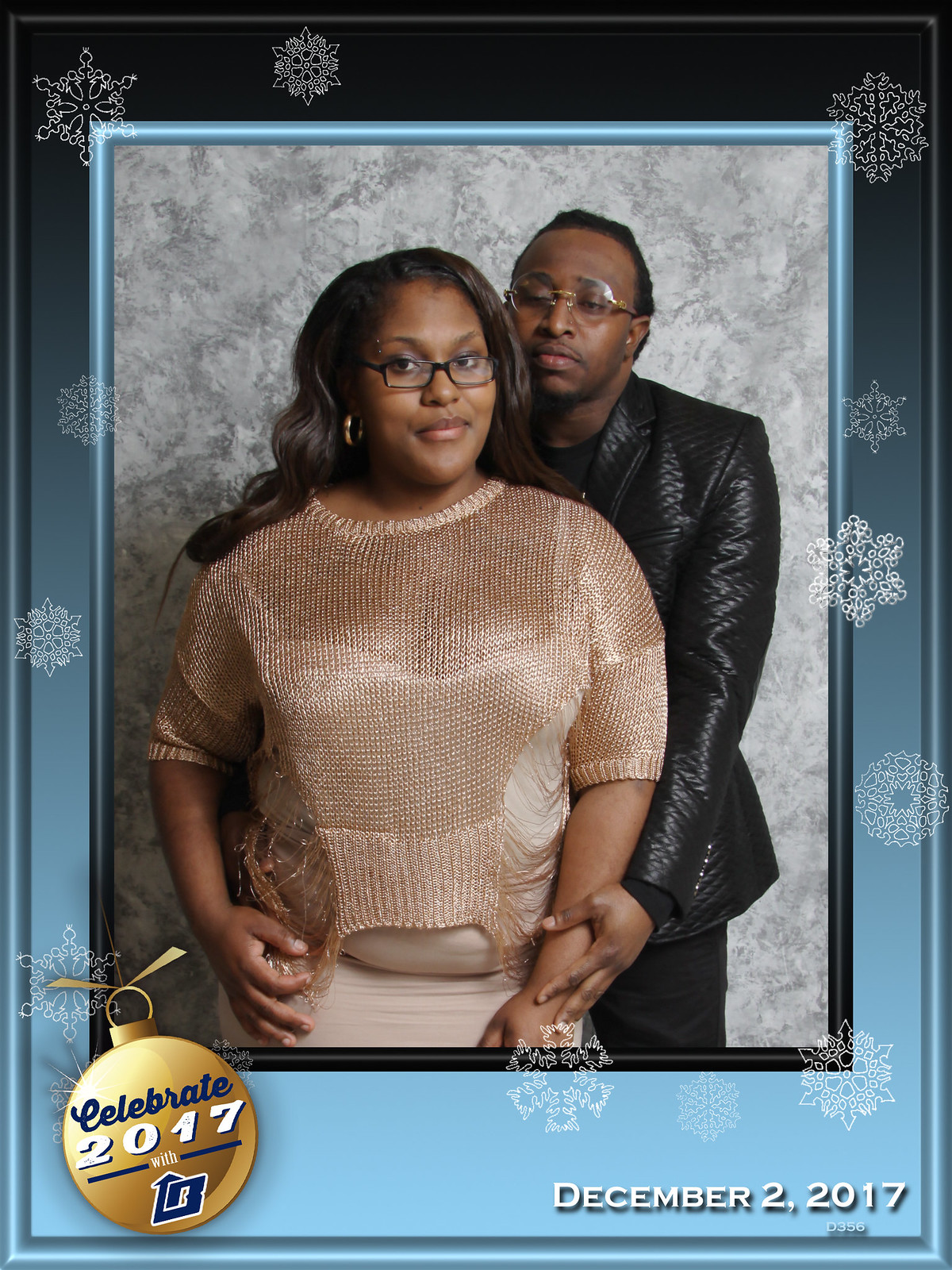The photograph features a festive scene framed with a vibrant blue border adorned with stylized cartoon snowflakes. In the bottom left corner of the border, a 2D Christmas ornament graphic showcases the blue text "Celebrate" above the white text "2017," accompanied by a logo resembling an arrow and a bee at the bottom of the ornament. In the bottom right corner of the entire image, the date "December 2, 2017" is inscribed in white text alongside the code "D356."

The central photograph captures a man and a woman posing together. The woman stands in the foreground, wearing a metallic sequin short-sleeve shirt paired with a tan-colored skirt. Her accessories include black-rimmed glasses and gold hoop earrings. Positioned behind her, the man is dressed in a black jacket and black pants, completing the ensemble. The festive border and holiday elements underscore the celebratory mood of the moment captured on December 2, 2017.